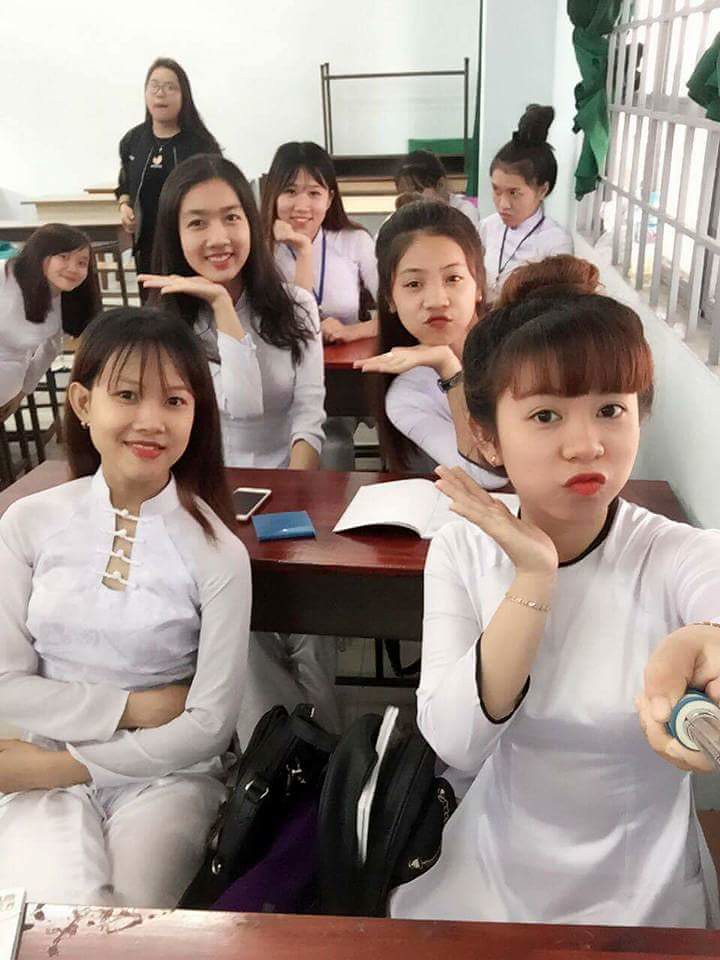This image features a selfie taken in a school setting, capturing a lively group of nine young Asian women standing at wooden desks. They are all dressed in white, creating a cohesive and coordinated appearance. The background includes a teacher, identifiable by her dark t-shirt, jacket, and glasses, who stands out amongst the students. The classroom's whitewashed walls, metal-barred windows with open green tapestries, and well-maintained brown desks suggest an organized and bright learning environment. 

In the forefront, a girl holds a selfie stick to capture the moment, and the expressions range from dramatic poses, with several girls flaring their palms underneath their chins, to others simply smiling or crossing their arms. Notably, one girl in the back right appears upset, looking away from the camera, and another girl is partially obscured by someone in front of her. Additionally, some benches are seen stacked upside down in the background, further enhancing the sense of a bustling classroom scene.